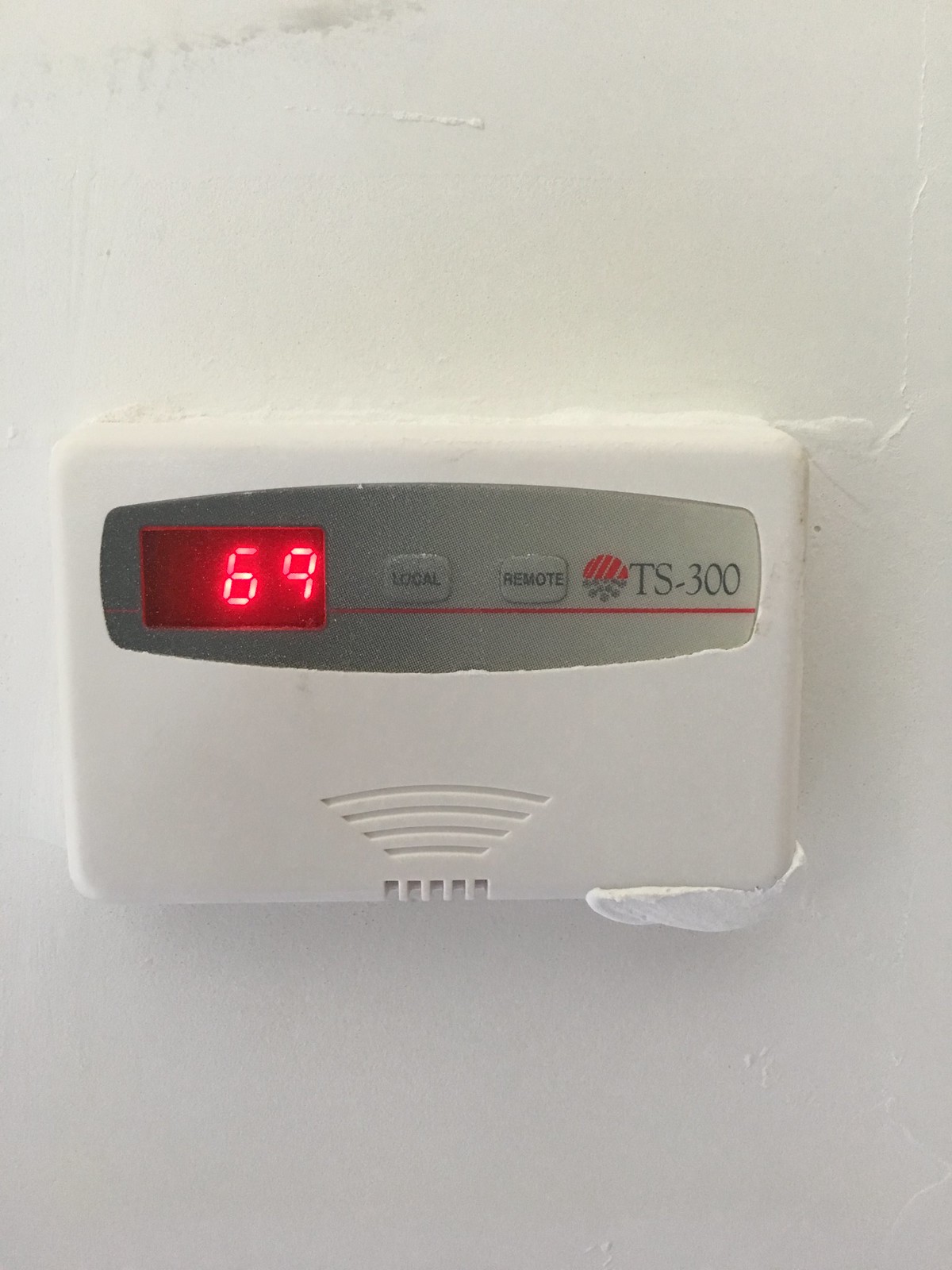This photograph showcases a section of a white wall with several notable details. At the top center of the image, there is a small grey dot accompanied by a smudged grey line beneath it. Further down, the wall features a subtle white bump forming a line, with another smaller bump to the right, adding texture.

Prominently displayed on the wall is a white thermostat. The bottom of the thermostat appears to be adorned with a white clay-like substance. It features five small square cutouts along its bottom edge. Above these cutouts are four distinct horizontal lines. The top portion of the thermostat houses a grey screen. 

To the left of this screen is a black display showing the number "69" in digital numerals. Adjacent to this display is a red horizontal line. Below the screen, there are two buttons labeled "OCAL" and "Remote," respectively. Additionally, a small red circle bearing the label "TS-300" is positioned near these buttons. 

The photograph meticulously captures these intricate details, painting a vivid picture of the wall's and thermostat's characteristics.